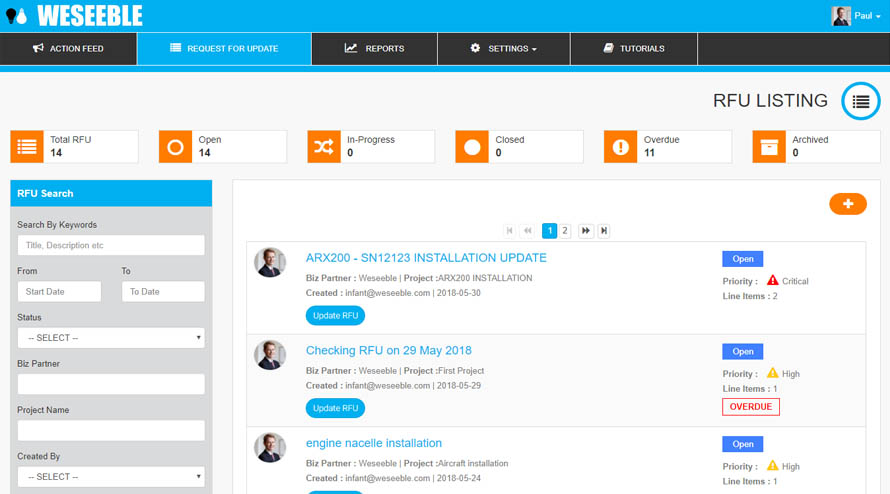This screenshot captures a detailed view of the WESEBLE website, showcasing its interface elements against a white background. At the top, a light blue banner spans horizontally across the screen. The header section prominently displays the website's name, "WESEBLE," alongside its unique icon featuring two light bulbs—one black and upright, the other white and inverted. 

In the top-right corner, a profile picture labeled with the name "Paul" and an accompanying arrow are visible. Below the banner, specific headers categorize the site’s main functions: Action Feed, Request for Update, Reports, Settings, and Tutorials. "Request for Update" is highlighted in blue, indicating the currently selected section.

The primary content area is organized methodically. Five distinct orange icons are evenly distributed across the page, each indicating different statuses: Total RFU, Open, In Progress, Closed, Overdue, and Archived. Positioned centrally above these icons, a blue-outlined circle features the label "RFU listening" to its left.

To the left of the main section (bottom left area of the image), a vertical grey box titled "RFU Search" provides various search filters, allowing users to refine their queries by Keywords, From and To dates, Status, Business Partner, Project Name, and Created By.

Within the central area of the screen are three installation updates, each linked with a profile picture of the same individual. Each update has an "Open" button on its right side, while the middle update is distinctly marked with a red-bordered box that reads "Overdue." The layout and elements of this screenshot succinctly depict the functional and navigational aspects of the WESEBLE website.